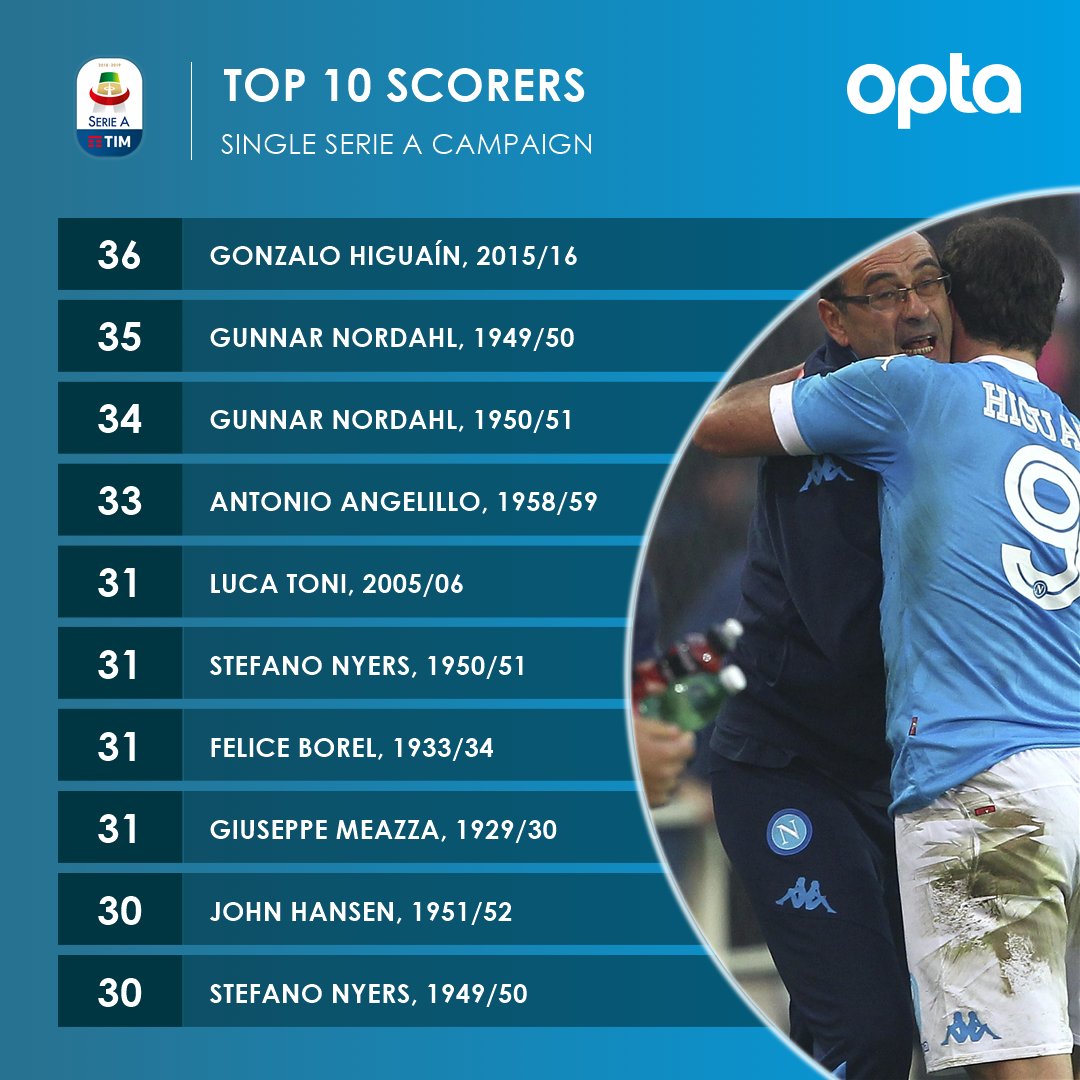The image displays a detailed scorecard highlighting the top 10 scorers in a single Serie A campaign. The focal point on the right features a soccer player wearing a blue short-sleeved t-shirt with white trim around the arms and collar. His name is partially visible as "H-I-G-U-A," likely representing Gonzalo Higuaín. The number nine adorns the back of his jersey, and he is sporting white shorts that are stained with grass.

Above the player, the word "Opta" is printed in white. The top left corner of the scorecard reads "Top Ten Scorers in a Single Serie A Campaign," supplemented by a Serie A TIM emblem. The list below ranks the players by their goal tally and season:

1. **Gonzalo Higuaín** - 36 goals (2015/16)
2. **Gunnar Nordahl** - 35 goals (1949/50)
3. **Gunnar Nordahl** - 34 goals (1950/51)
4. **Antonio Angelillo** - 33 goals (1958/59)
5. **Luca Toni** - 31 goals (2005/06)
6. **Stefano Nyers** - 31 goals (1950/51)
7. **Felice Borel** - 31 goals (1933/34)
8. **Giuseppe Meazza** - 31 goals (1929/30)
9. **John Hansen** - 30 goals (1951/52)
10. **Stefano Nyers** - 30 goals (1949/50)

This scorecard recognizes the outstanding performance of these players, with Gonzalo Higuaín leading the list for the 2015/16 season.